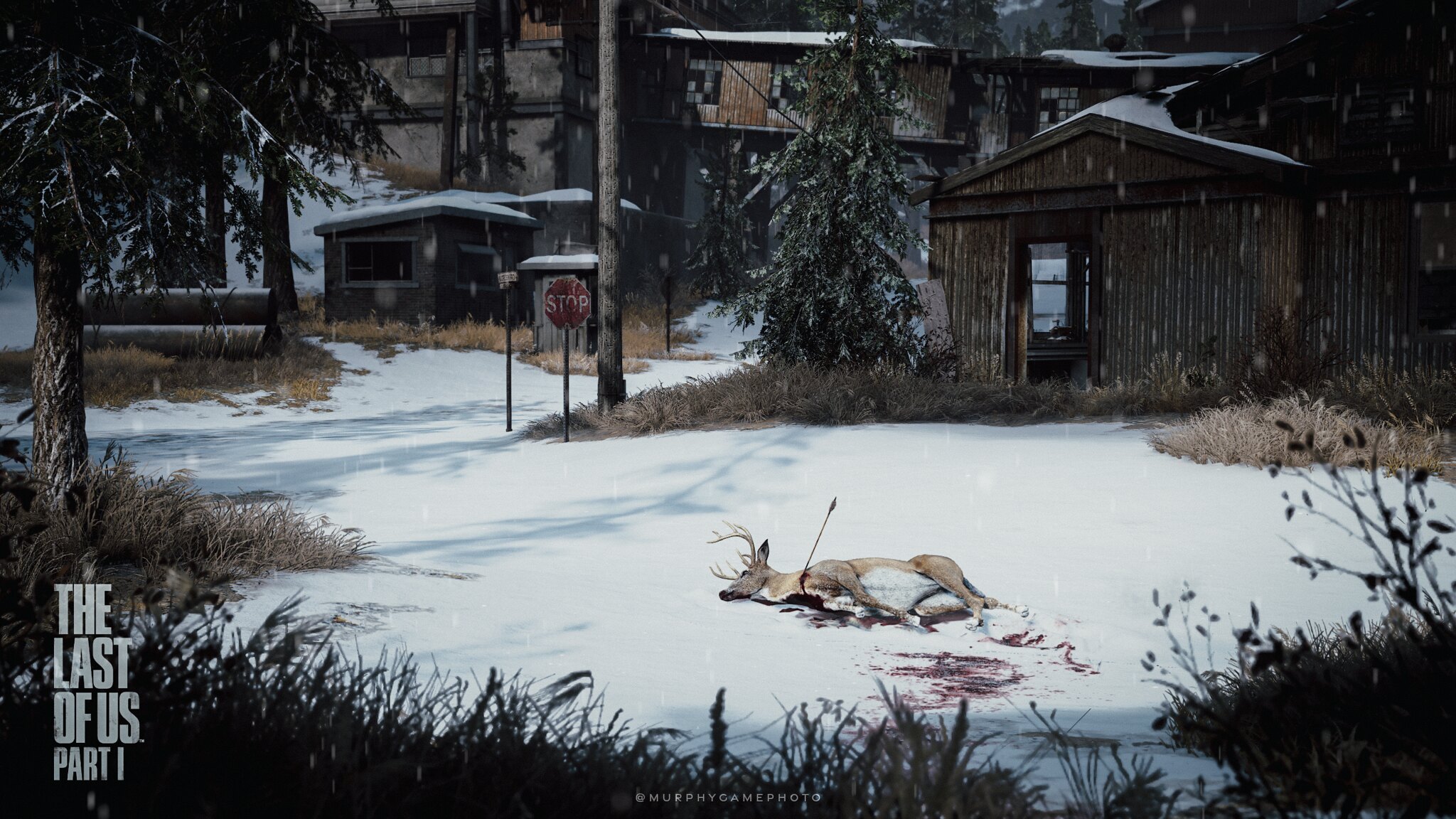This detailed rendering depicts a quaint village nestled amid winding roadways and pathways. The ground is blanketed in snow, which contrasts against the surrounding brownish-yellow grass. In the foreground, a lifeless deer lies on its side, an arrow protruding from its neck. Its antlers, adorned with three points each, add to the somber scene. Notably, the image bears the title "The Last of Us Part One" in white text on the bottom left, while "Murphy Game Photo" is inscribed in smaller white print along the bottom edge, lending a sense of authenticity and context to the scene.